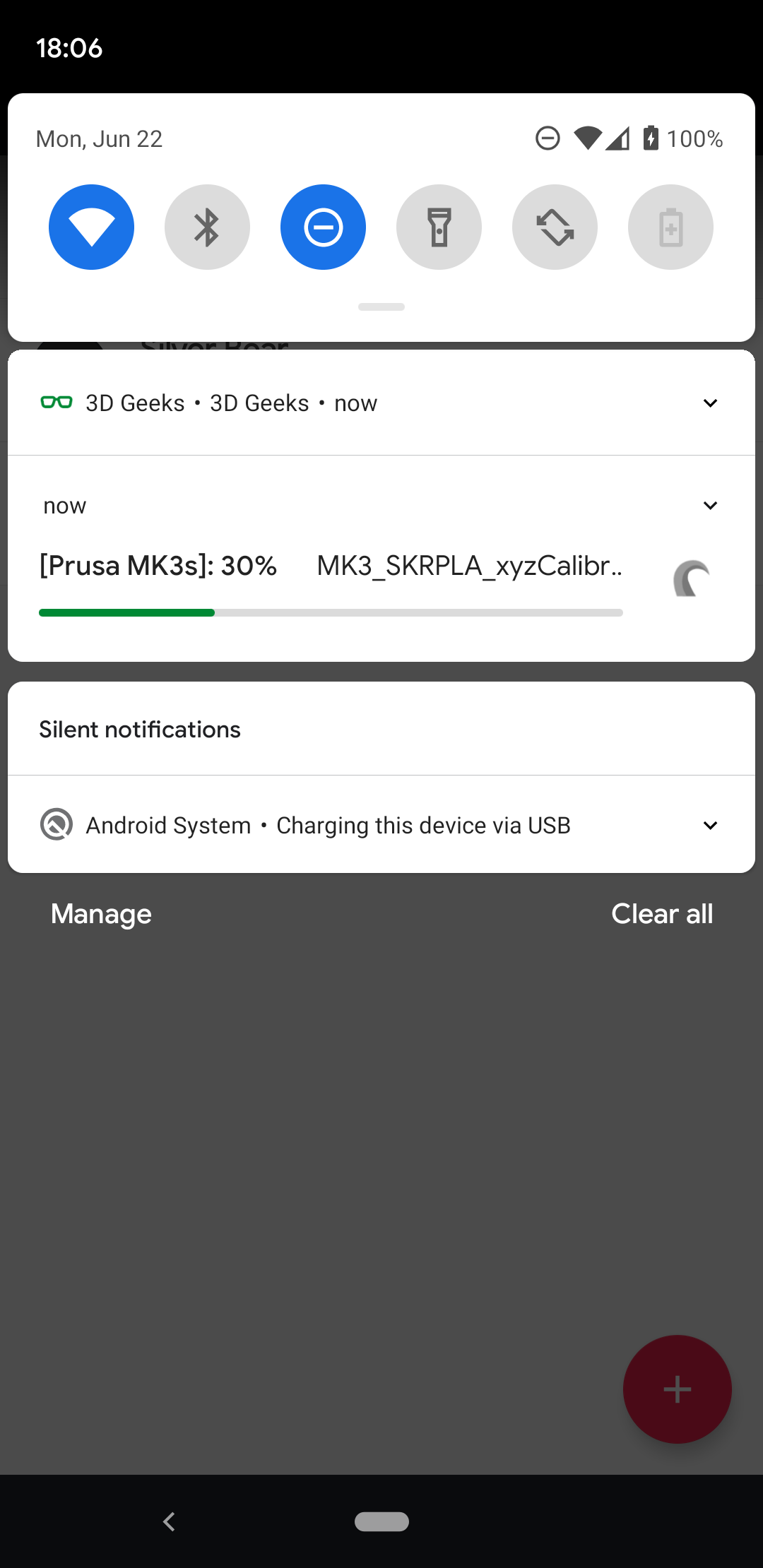This is a detailed descriptive caption for an Android phone screenshot:

"The screenshot of an Android phone displays a status bar at the top showing the time as 18:06. Below the time, there is a white box on the left side indicating the date as June 22nd. To its right, there are several icons including a 'Do Not Enter' symbol, Wi-Fi symbol, signal strength indicator, and a battery icon showing 100% charge. Below this, there is a series of quick setting buttons: a blue button for Wi-Fi, a grey button for Bluetooth, a blue button for 'Do Not Disturb,' a grey button for the flashlight, a grey button for mobile data, and a grey button representing battery saver.

Further down, there is an icon of green glasses associated with the '3D Geeks' app. The display reads '3D Geeks Now', followed by 'Now' in parentheses and details such as 'Mk3S 30%' and 'Mk3SKRPLAXYZ.' Beneath this, a green progress bar is visible. 

The next section of the screen lists a box labeled 'Silent Notifications,' with a notification stating 'Android system charging this device for USB.' Finally, at the bottom, there is a grey box containing partial text that starts with 'Marriage. If you are.' with a red plus button located at the very bottom of the screen."

This caption provides a comprehensive description of the various elements visible in the screenshot.